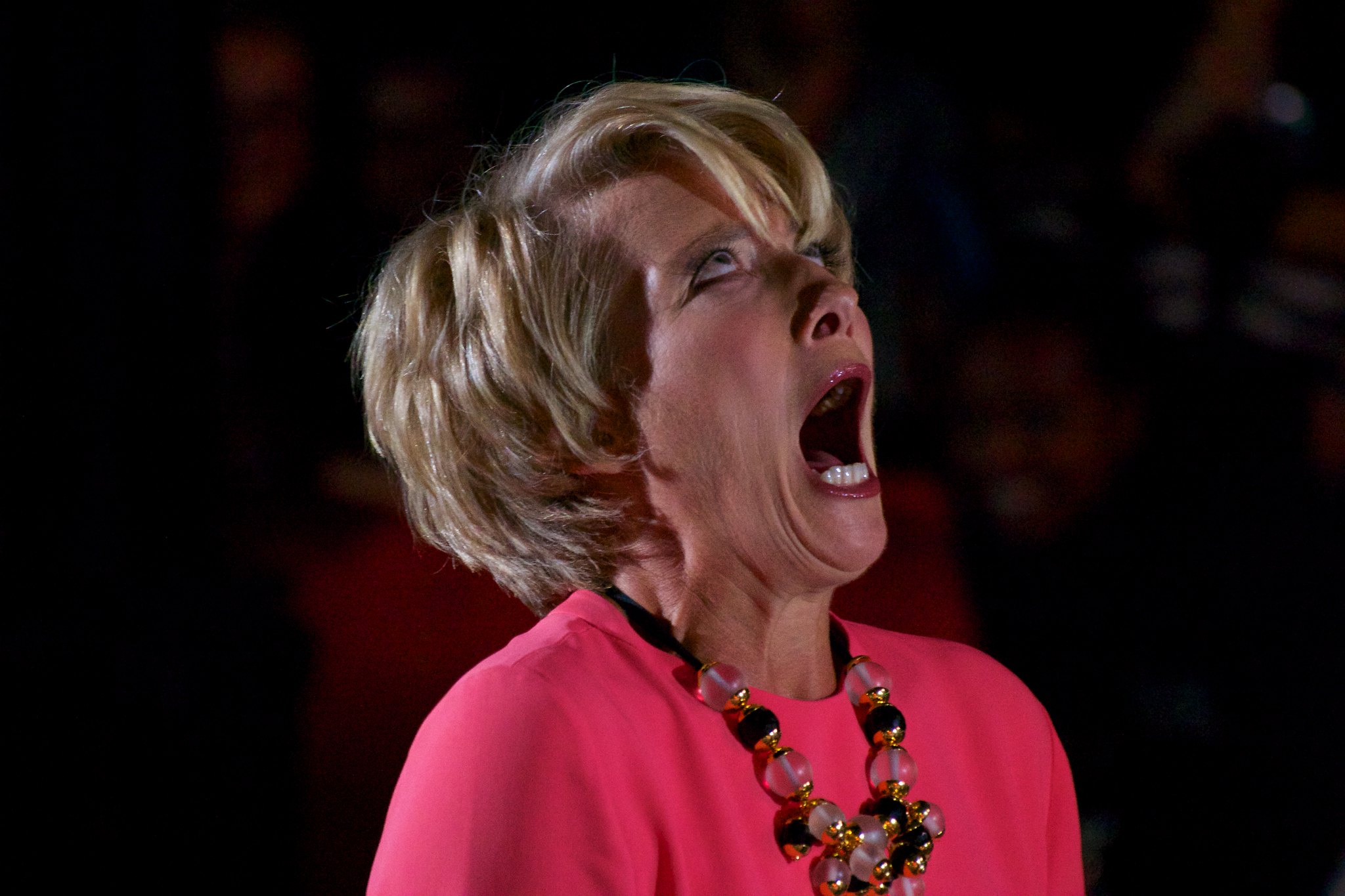The image is a medium close-up shot of a woman who appears to be in her 50s with short, wavy blonde hair, wearing a pink top. She has a necklace made of alternating black and clear glass-like beads. The woman is looking up with her mouth open wide, suggesting she might be yelling, shouting, gasping, or swimming. Her eyes seem rolled back into her head, adding a sense of intensity to her expression. The background is predominantly black, with a few extremely blurred outlines of people's faces visible, lending an ambiguous and dramatic atmosphere to the scene. The woman has pinkish lipstick and a striking presence, making the image captivating and evocative.